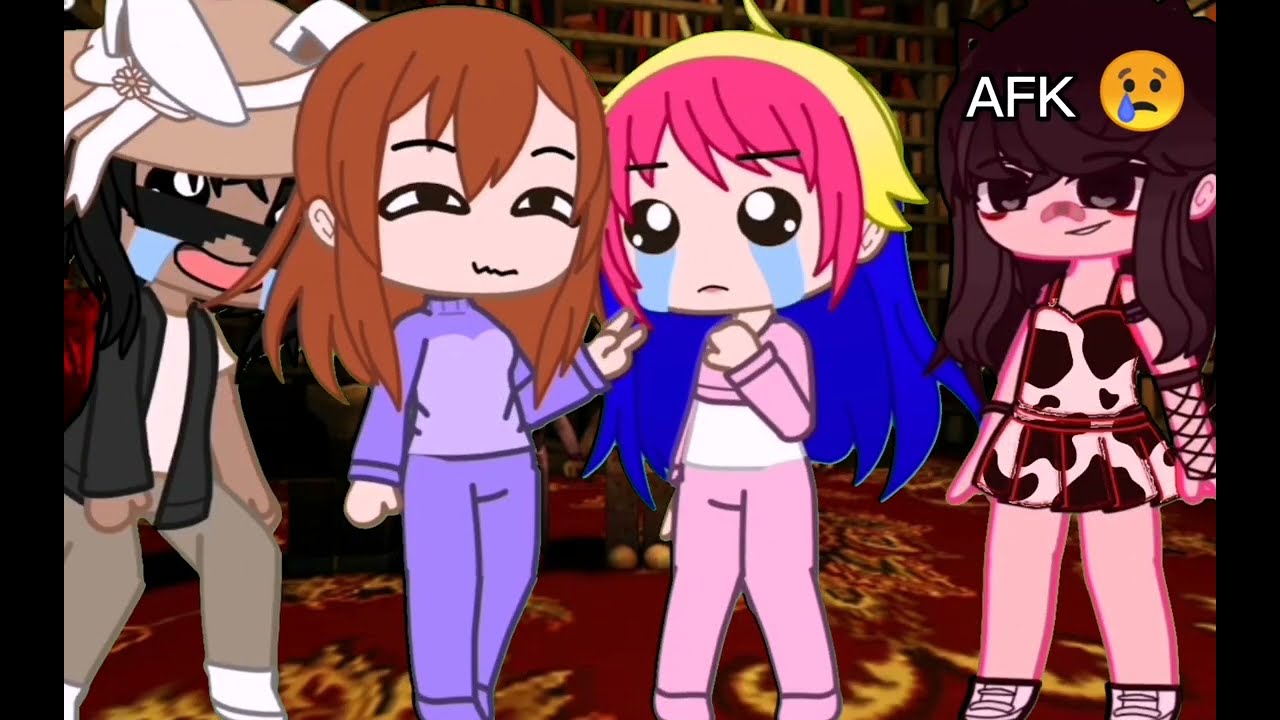The digital cartoon image features four distinct characters against a backdrop that hints at a club scene. Starting from the left, the first character is wearing a beige hat with rabbit ears, a short-sleeved t-shirt under a black open vest, and beige pants. This character also sports dark hair and sunglasses, with tears flowing down their face. The second character appears to be a woman with red hair dressed in a two-piece purple sweatsuit. She is making a peculiar gesture with her left hand and has a squiggly line for a mouth, indicative of a mixed expression. The third character stands out with her multicolored hair—pink, yellow, and blue—and is visibly crying. She is clad in a pink sweater and matching pink pants, her posture slightly inward with knees pointed together. Lastly, on the far right, there is a girl with long brown hair and bangs, dressed in a cow print miniskirt with a pleated design. She completes her look with high-top sneakers and arm nets, and an "AFK" label with a sad emoji is positioned above her shoulder.